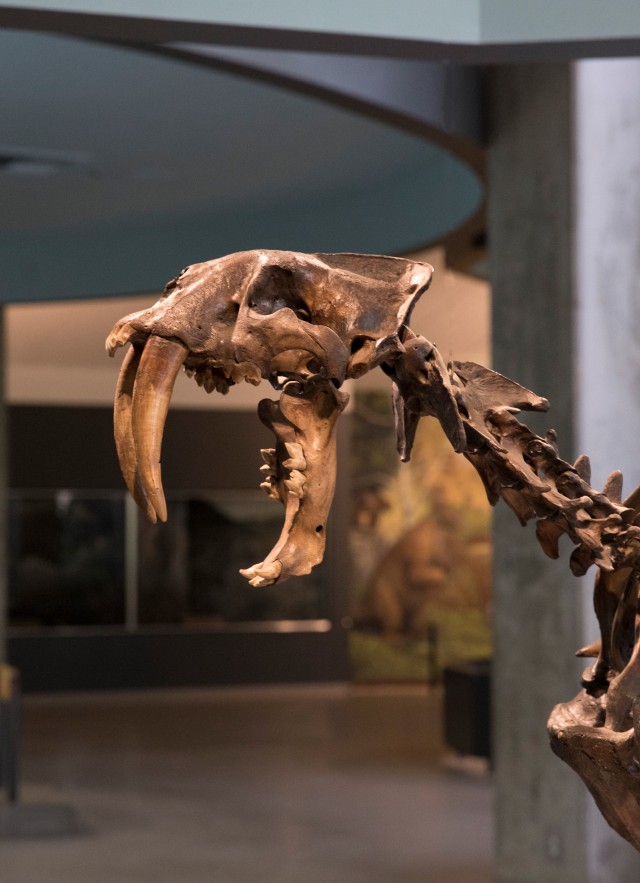This detailed, vertically rectangular full-color photograph, taken indoors using artificial light, captures the partial skeleton of a saber-toothed tiger (also known as a saber-toothed lion) prominently displayed in a museum setting. The skeleton appears in the lower right-hand corner, extending towards the center left of the image, showcasing its distinctive brown bones. The saber-toothed tiger's head is arched dramatically, displaying its wide-open jaw fitted with impressively long front fangs, estimated to be at least eight inches in length. The vertebrae of the neck are clearly visible, presenting at least five darkened neck vertebrae before the chest area begins, from where the rest of the body trails off out of the photograph.

The background is somewhat out-of-focus, providing a muted, grayish-white wall and a gray floor that set the scene without dominating the image. Further back, one can discern a couple of display cases, an artwork featuring a dinosaur to the right, and a larger mural containing dinosaur illustrations. The setting is further described with a circular blue ceiling and additional museum displays, indicating the educational and historical ambiance of the location. This fusion of details from multiple descriptions offers a comprehensive view of the scene, drawing attention to the awe-inspiring skeletal remains while contextualizing its museum environment.